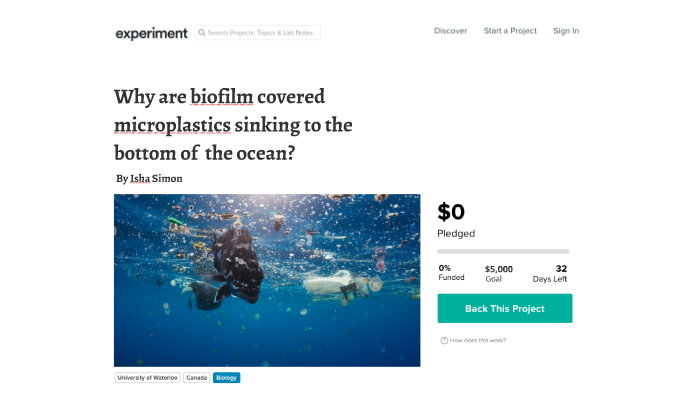This is a detailed screenshot of an experimental project on a crowdfunding website similar to Kickstarter. In the top left corner, in all lowercase letters, the word "experiment" is displayed. To its right, there is a long search bar. On the top right side of the screen, there are menu options labeled "discover," "start a project," and "sign in."

Towards the bottom right, there are numerical details indicating the financial progress of the project. A gray line stretches horizontally beneath the pledged amount section. Below this line, the statistics show "0 dollars pledged," "0% funded," a "5,000 dollar goal," and "32 days left." Immediately under these details, there is a green bar with white text that reads "back this project."

On the left side of the screenshot, the headline "Why are biofilm-covered microplastics sinking to the bottom of the ocean?" is prominently displayed. This project is by Isha Simon. Below the headline, a rectangular photograph with a horizontal orientation captures the view from beneath blue water, showing a significant amount of trash floating on the water's surface.

Underneath the photograph, there are three clickable buttons. The first button says "University of Waterloo," the second one says "Canada," and the third one, which is blue, appears to say "biology," though it is not entirely clear.